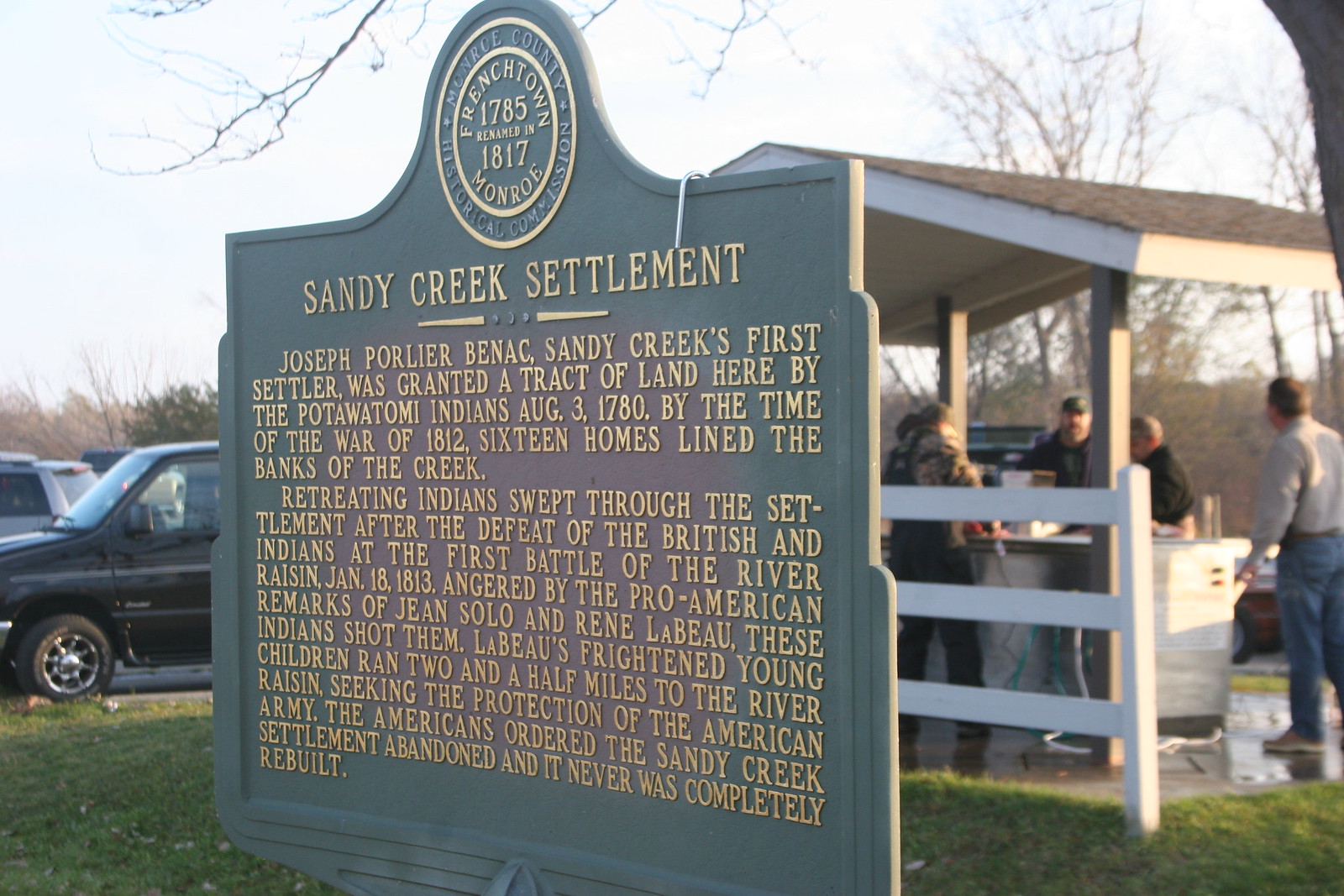The image depicts an outdoor scene centered around a historical sign placed on a well-maintained grassy area. The sign, with a green background and a round emblem at the top, provides a detailed account of the Sandy Creek Settlement. It reads: "Sandy Creek Settlement. Joseph Poirier Bennett, Sandy Creek's first settler, was granted a tract of land here by the Potawatomi Indians on August 3rd, 1780. By the time of the War of 1812, 16 homes lined the banks of the creek. Retreating Indians swept through the settlement after the defeat of the British and Indians at the First Battle of the River Raisin, January 18th, 1813. Angered by the pro-American remarks of Jane Sobo and Renee LeBow, these Indians shot them. LeBow’s frightened young children ran two and a half miles to the River Raisin, seeking the protection of the American Army. The Americans ordered the Sandy Creek Settlement abandoned, and it was never completely rebuilt."

The top of the sign features a circular emblem with golden borders and inscriptions. The outer ring says "Frenchtown, 1785," and the inner ring says "Reclaimed in 1817," with "Monroe" written underneath. Faint blue lettering is also present but is difficult to read.

Behind the sign, a white-roofed gazebo stands, characterized by an arched roof and supported by gray poles. Underneath the gazebo, four to five people, some wearing blue jeans, are gathered around a silver container on a concrete surface. The background shows a black van with a chrome wheel parked to the right, leafless trees, and a sky that transitions from white to a hint of blue on the left side.